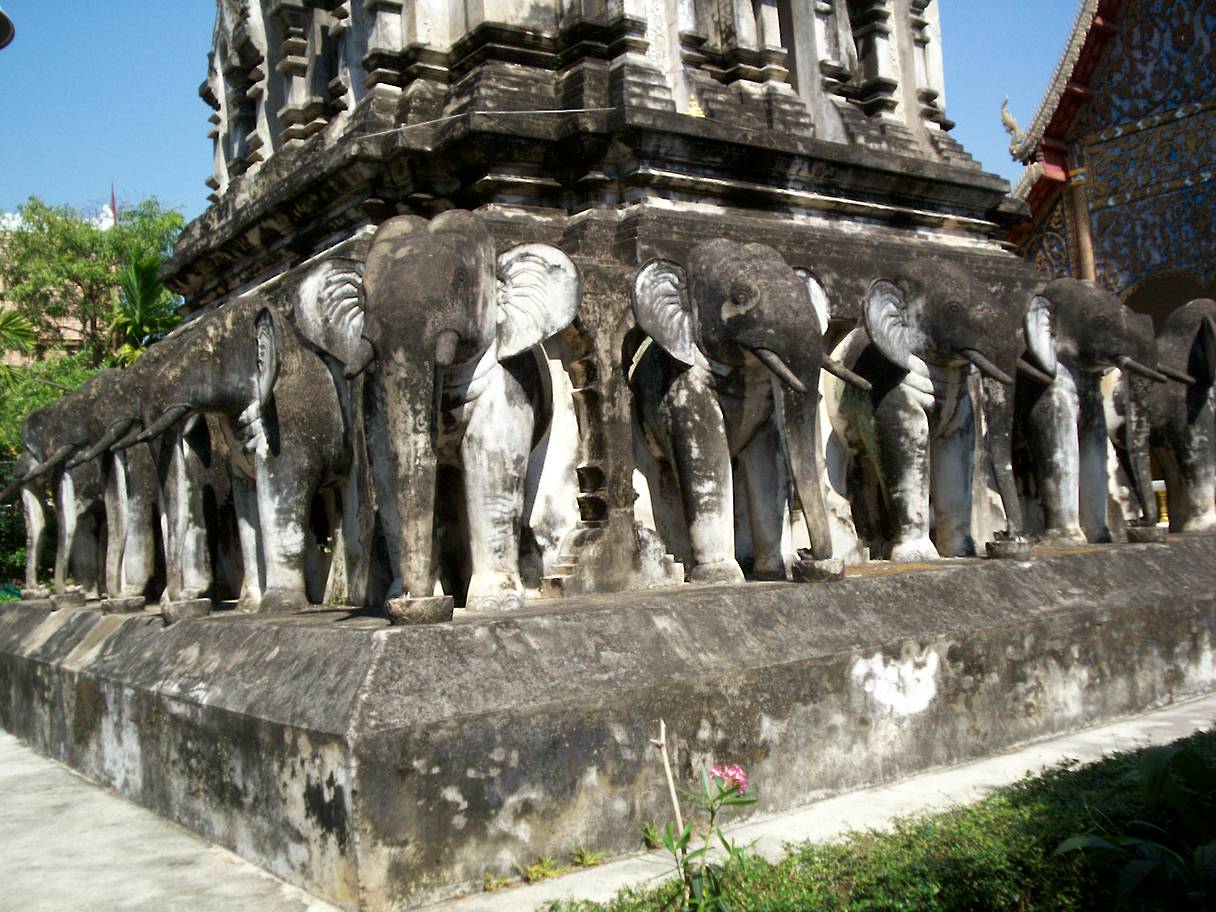The image features an ancient, weathered stone monument, possibly a shrine or temple, supported by numerous intricately carved elephant statues. Each side of the large, heavy stone base is adorned with elephants, some with their tusks resting in stone bowls, showing significant signs of aging with dark grime and black growth. The elephants, originally white, now appear gray due to dirt and weather exposure over time. The base and the elephants are crafted from a grayish-white, concrete-like material, and they support tall, clustered pillars, forming the main structure of the monument. Surrounding the monument is an off-white concrete walkway, adjacent to patches of green grass, featuring a small pink flower. In the background, a finely detailed, ornate wooden building with blue insets and decorative borders stands, alongside dark brown and black structures and some palm-like trees, indicating a tropical setting. Overhead, a bright blue sky with no clouds completes the scenic, historical panorama.